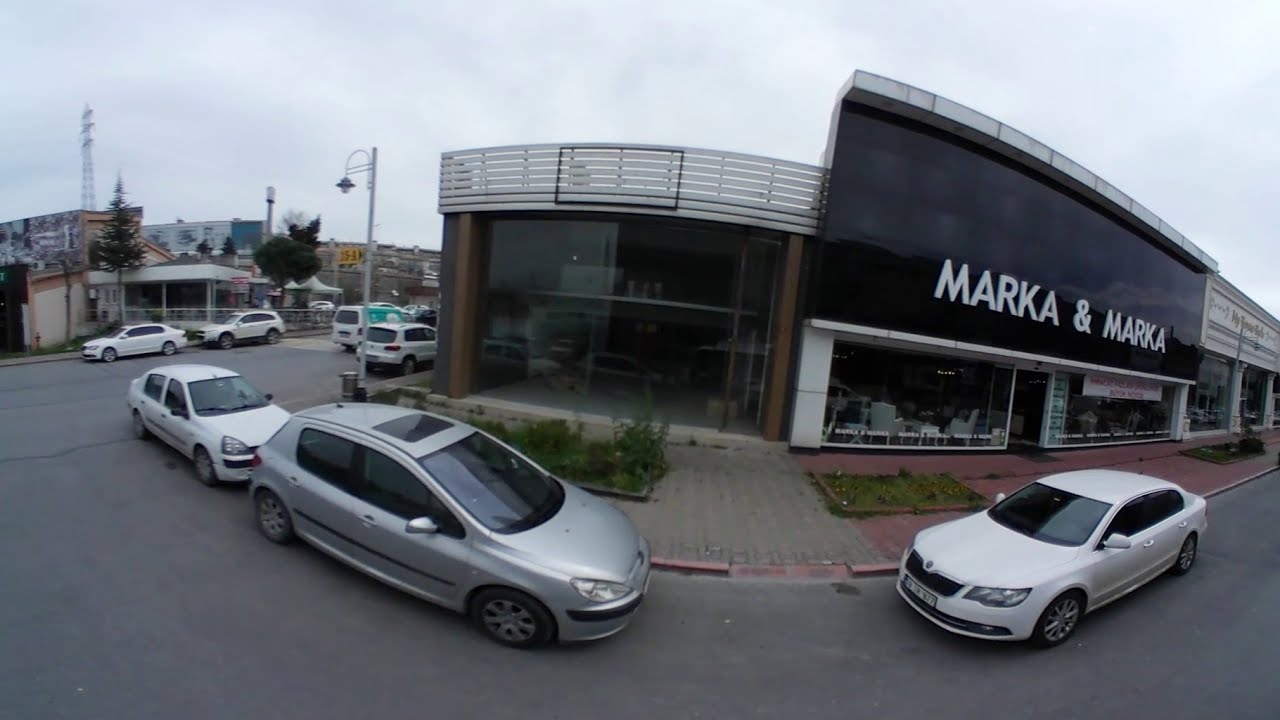In this detailed image of a city street, framed in a horizontal rectangular shape, the foreground prominently features a two-story building with a modern design. On the left side of the building, a large expanse of glass fronts the structure, giving a clear view into what appears to be an interior populated with chairs, suggesting its identity as a potential furniture store or restaurant. Dominating the upper section of the building's front is a large black metal sign that extends above the roofline, emblazoned with "Marca and Marca" in bold white letters.

The scene extends to the right of this building, where another store is visible but its sign remains unclear. In front of the buildings, several cars are parked along a red and gray brick sidewalk adorned with rectangular planters that host patches of greenery, adding a touch of nature to the urban setting. The sidewalk continues to the left of the building, following the street that stretches into the distance past more parked cars and additional structures.

The street itself is depicted in a dark gray hue, complementing the overcast sky that blankets the scene in shades of gray and white, contributing to the overall dreary atmosphere, possibly indicating a winter day. Notably, the parking area in front of the building showcases a mix of mainly white cars, with a few gray ones interspersed. Light posts line the street, blending into the gray background. The presence of grass and trees with green foliage and brown branches adds contrast and life to the otherwise muted palette of the image.